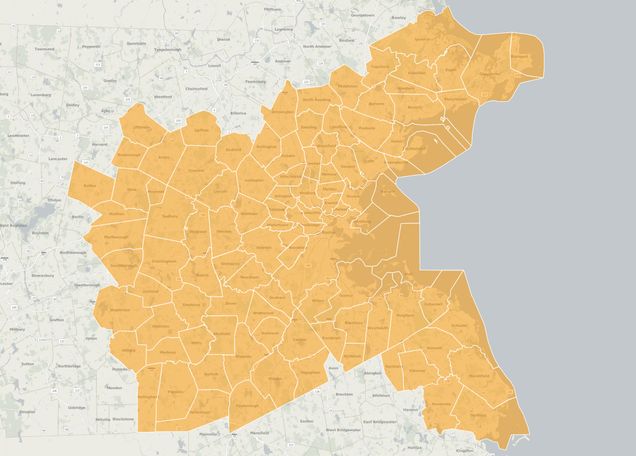The image portrays a map with a distinct focus on an area marked by various orange or mustard yellowish counties, suggesting it could represent a region within a state or country. These highlighted counties are centered on the map, surrounded by regions in cream or off-white tones to the left, signifying other counties or states. The far right side of the image is dominated by a dark gray color, possibly indicating a large body of water such as the sea or ocean. Despite the presence of labels on the map, they are unreadable due to the small and pixelated text. The map seems to illustrate both coastal and inland areas, with the orange counties serving as a focal point amidst the otherwise muted color scheme.